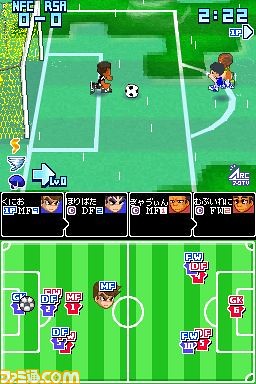The image is a screen capture from an animated, non-realistic soccer video game, likely from a mobile app. The game interface is vertically rectangular, and the top part features an animated soccer field with a yellow-netted goal on the left. The green grass field is marked with white lines and shows three little avatars actively engaged in play: the goalie, an African-American character, is positioned near the goal with a soccer ball at their feet, while two other avatars are running towards the ball from the right.

In the top left corner, there is a scoreboard displaying a 0-0 tie, with acronyms likely representing the team names. The top right corner indicates a remaining game time of 2:22. Below this main action, a banner with four black boxes seems to represent the players or their respective levels. At the very bottom is a horizontal rectangular section of the entire soccer field, providing a mini-map that shows the positions of all avatars on the field. The image also includes a small text in the bottom left corner, which appears to be a website URL, dzeio.com, perhaps indicating the game's origin.